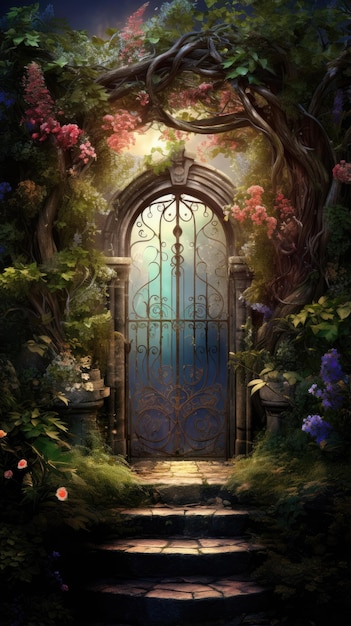The image captures an enchanting scene reminiscent of a fantasy realm. Central to the picture is an ornate metal gate ensconced underneath a beautifully overgrown stone archway. The gate, which features intricate floral patterns on its lower side and artistic loops above, is framed by multicolored vines and vegetation, showcasing hues of green, blue, and red intertwined with vibrant flowers. The stone archway leading up to it is accessible via four cobblestone steps that invite the viewer into this mystical setting. The archway itself, bathed in a mix of light and dark blues and whites, suggests an ethereal atmosphere. The overall ambiance hints at an inviting yet mysterious realm, as though the gate leads to a hidden garden or a secret, fantastical world, with a sky tinged in blue and white casting an almost magical light over the scene.